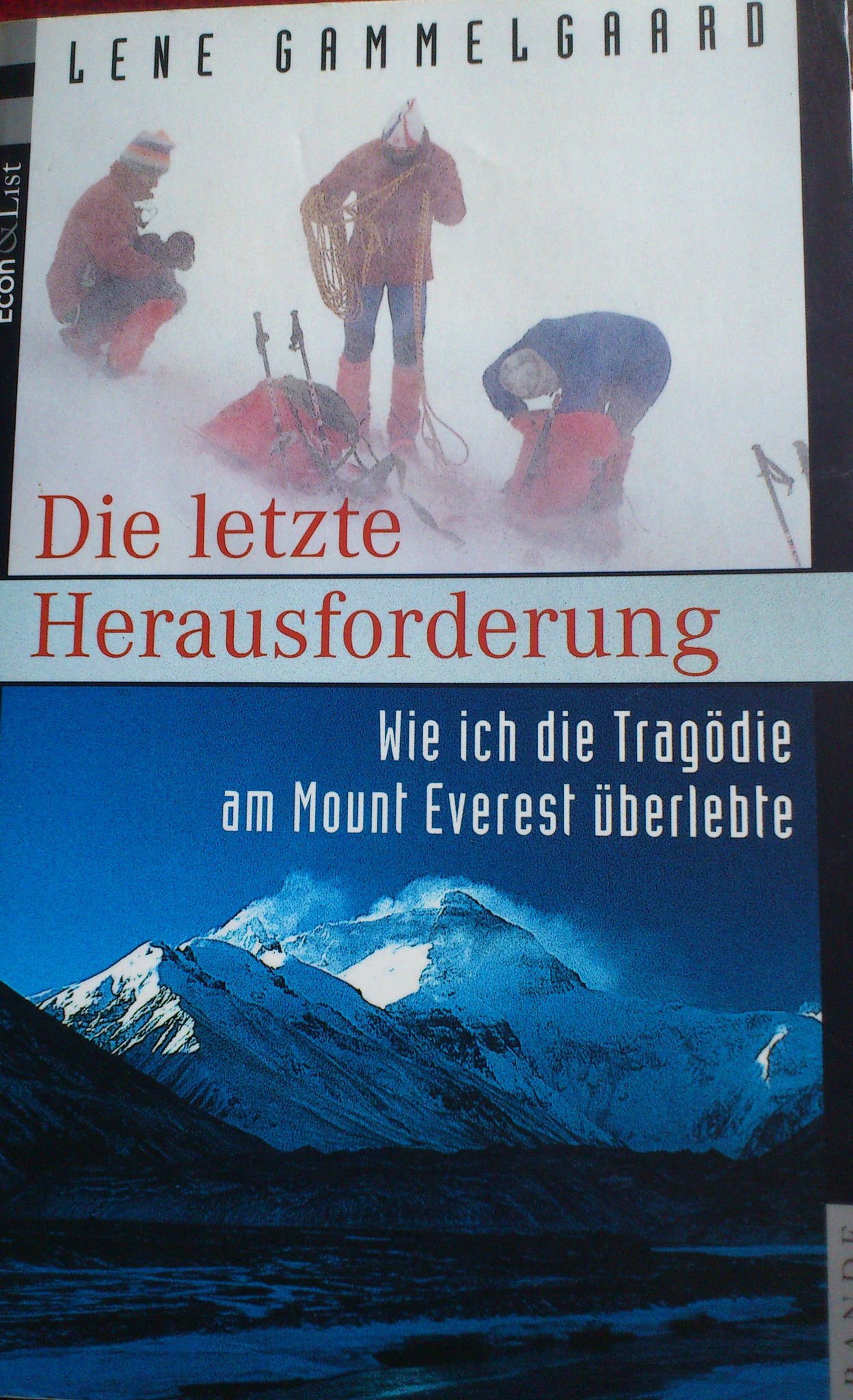The image is a vertically aligned rectangular cover, likely for a poster or book. The top part features a white background with the name "Lene Gammelgaard" written in bold black text. Below this, there’s an image of three individuals standing in a snowy landscape, equipped with winter gear including hats, jackets, and backpacks. The person in the middle is holding an orange extension cord, and a red tool is visible on the ground, highlighting their preparedness for a rigorous activity, possibly mountaineering or skiing. In the bottom left-hand corner of this snowy scene, the text "Die Letzte" is visible. Below this, another image showcases a large, snow-covered mountain against a predominantly blue background, with more flat, snow-covered terrain at the bottom. Bold red text across this image reads, "Herausforderung," while in the top right corner, white text spells out "Y-I-C-K-D-I-T-R-A-G-O-D-E-M Mount Everest, Uberlept." The clarity of the images is high, making the scene and text easily distinguishable.